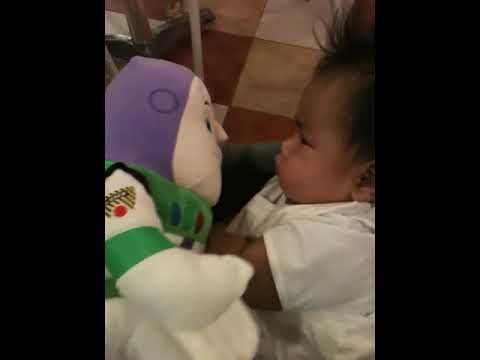This is a small square photograph with vertical black borders on either side, featuring a baby boy and a toy in the center. The baby, who appears to be of Asian or ethnic descent with slightly dark skin and black hair, is positioned to the middle right of the image. He is around three to six months old, wearing a white, short-sleeve top or possibly a onesie. The baby is captured in profile, gazing intently at a large toy positioned in front of him. Even though the baby doesn't hold the toy, his arm extends towards it. This toy, which is almost the same size as the baby, resembles a male character, possibly Buzz Lightyear from Toy Story. The toy is predominantly white with black eyes, a pointed nose, a purple seamless headpiece, and green accents including bands, shoes, and a collar. The toy's chest also features colorful buttons and an Asian logo on its right arm, depicting a red sun beneath slanted black stripes. The vivid details create a captivating snapshot of curiosity and wonder.